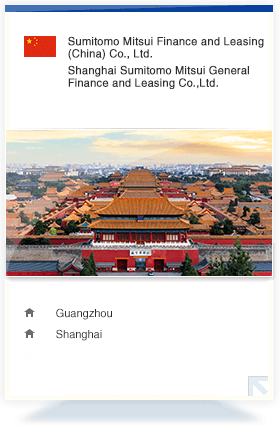The website showcases an aerial photograph of an imposing structure, identified as being located in Shanghai. This grand edifice, which appears far too large to be a mere house and more akin to a palace, features a distinctive architecture with a brown, steeply pointed roof and red exteriors. In front of the building stands a retaining wall, predominantly white with bluish-gray and red hues. The backdrop of the image reveals an urban landscape, suggesting the presence of a city behind the primary structure.

The top of the web page includes a blue navigation bar, highlighted by a red square adorned with a gold star and additional gold embellishments. On the upper left corner, the text reads "Tsunamido Mitsu Finance and Leasing China Company Limited, Shanghai Tsunamido Mitsu General Financing and Leasing Company Limited," repeated almost verbatim.

Below the photograph, the words "Guanzhou" and "Shanghai" are displayed, each accompanied by a home icon, implying navigational options. The entire content is shown on what seems to be a monitor, as evidenced by a shadow at the bottom, indicative of a stand or screen edge.